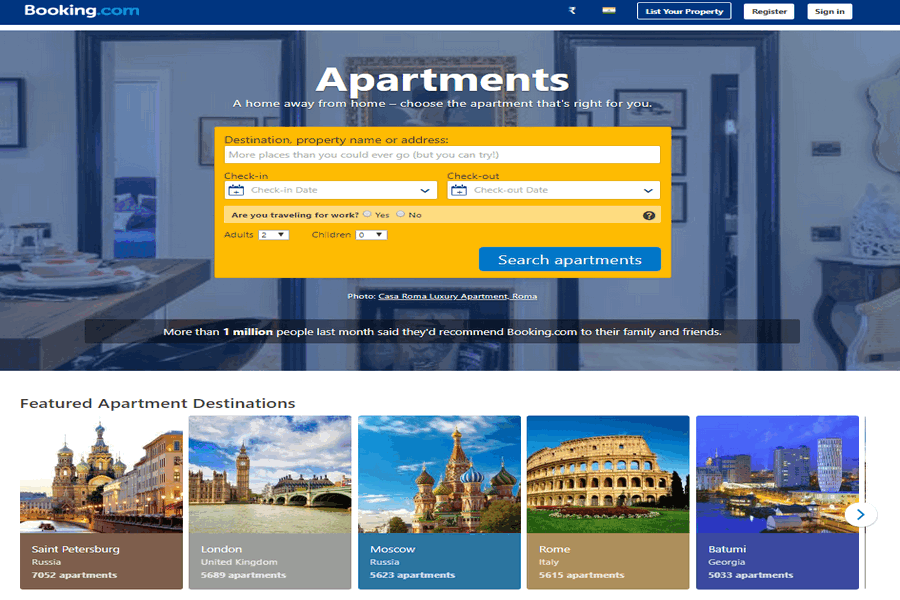The image showcases a Booking.com webpage designed for apartment reservations. The top portion features a blue background with the Booking.com logo prominently displayed; "Booking" is in white, while ".com" is in blue. Adjacent to the logo is a small white icon, followed by a white box labeled "List Your Property," along with "Register" and "Sign In" buttons.

Below this header is a navigation strip, under which lies a large photograph of an apartment. Overlaid on the image in white text are the words "Apartments: A Home Away from Home. Choose the apartment that's right for you."

Dominating the center of the page is a vibrant yellow search box. Inside this box are several interactive elements to enter booking details:
- A field labeled "Destination, property name, or address" followed by a large search box.
- "Check-in" and "Check-out" fields, each with a white box, a blue calendar icon, and a drop-down arrow.
- A question asking, "Are you traveling for work?" with a yellow background, featuring "Yes" and "No" options and a black circle with a question mark.
- Dropdowns for the number of "Adults" (set to 2) and "Children" (set to 0).
- A prominent blue "Search Apartments" button.

Below the search functionality, there is a testimonial statement: "More than one million people last month said they'd recommend Booking.com to their family and friends."

The remaining part of the webpage features a white background with a section titled "Featured Apartment Destinations," listing prominent cities including St. Petersburg, Russia; London; Moscow; Rome; and Batumi, Georgia.